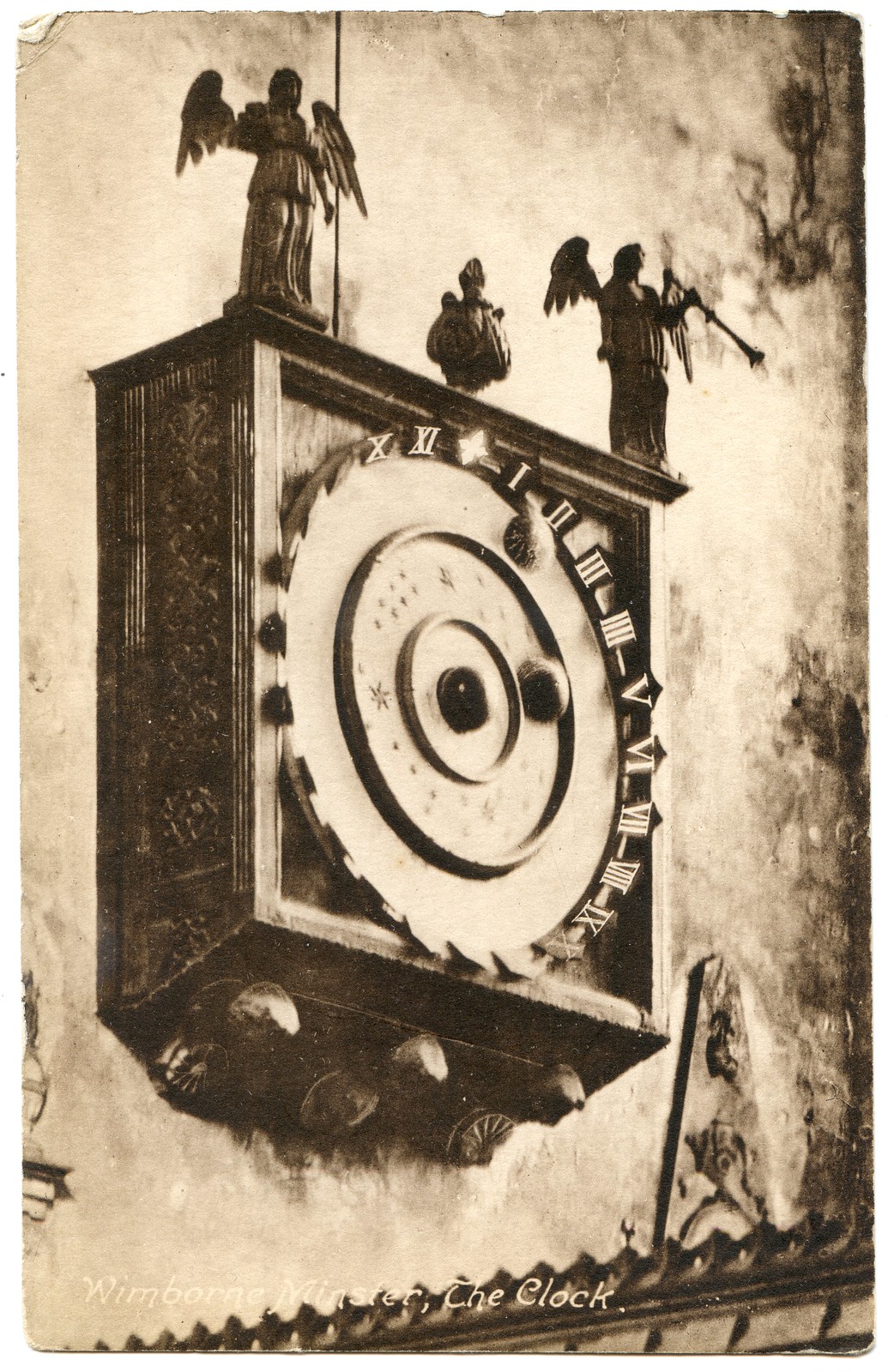The image is a faded, old black-and-white photograph showing an ornate, square clock from Wimborne Minster, labeled "Wimborne Minster, The Clock." The clock is set in what appears to be a wooden housing adorned with intricate designs along the sides and bottom. Although the photograph quality is poor, several details are discernible. The clock face, encircled by Roman numerals, features a large central gear and multiple inner circles. These circles depict celestial imagery, including stars and three planets, one of which points to the number two. At the top of the clock, two angel figurines holding horns flank a central, shorter figurine resembling a bishop. The background suggests the clock is mounted on a decorated wall, possibly featuring wallpaper or ornate trim.